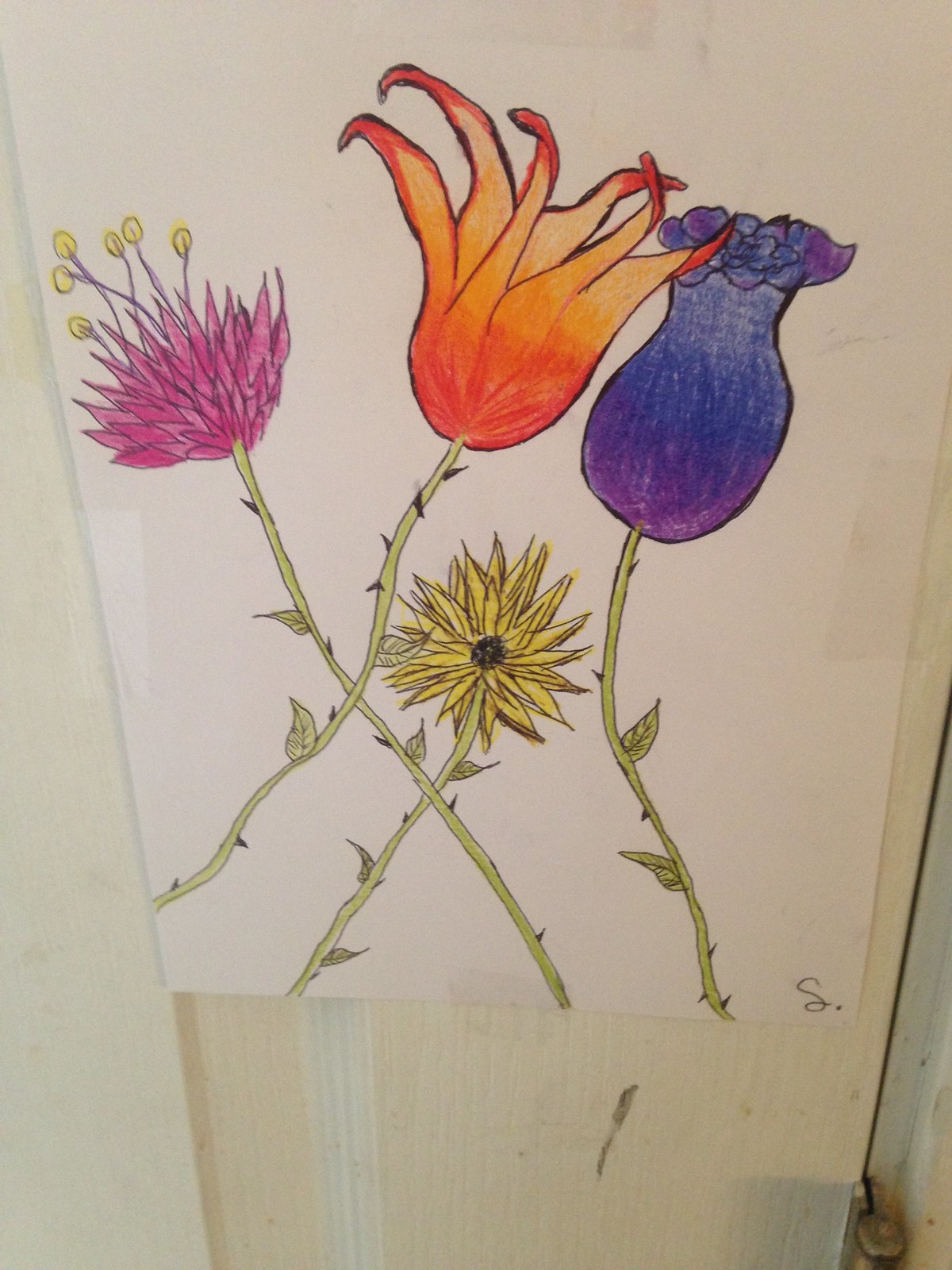The image is an intricate, hand-drawn and colored illustration of various types of flowers. At the center of the drawing is a prominent yellow flower, likely a sunflower, radiating a vibrant and cheerful hue. To the left, there is a striking bright pinkish-purple flower with delicately shaped petals, surrounded by small yellow blossoms that add a touch of charm to the composition. Adjacent to these is a fiery orangey-red flower with long, elegant petals that resemble flames. Beside this, a smaller, violet-purple flower appears to be in the early stages of blooming, tightly closed and full of potential. All the flowers are set against lush green stems, some adorned with tiny thorns and leaves that enhance the natural and lively feel of the artwork.